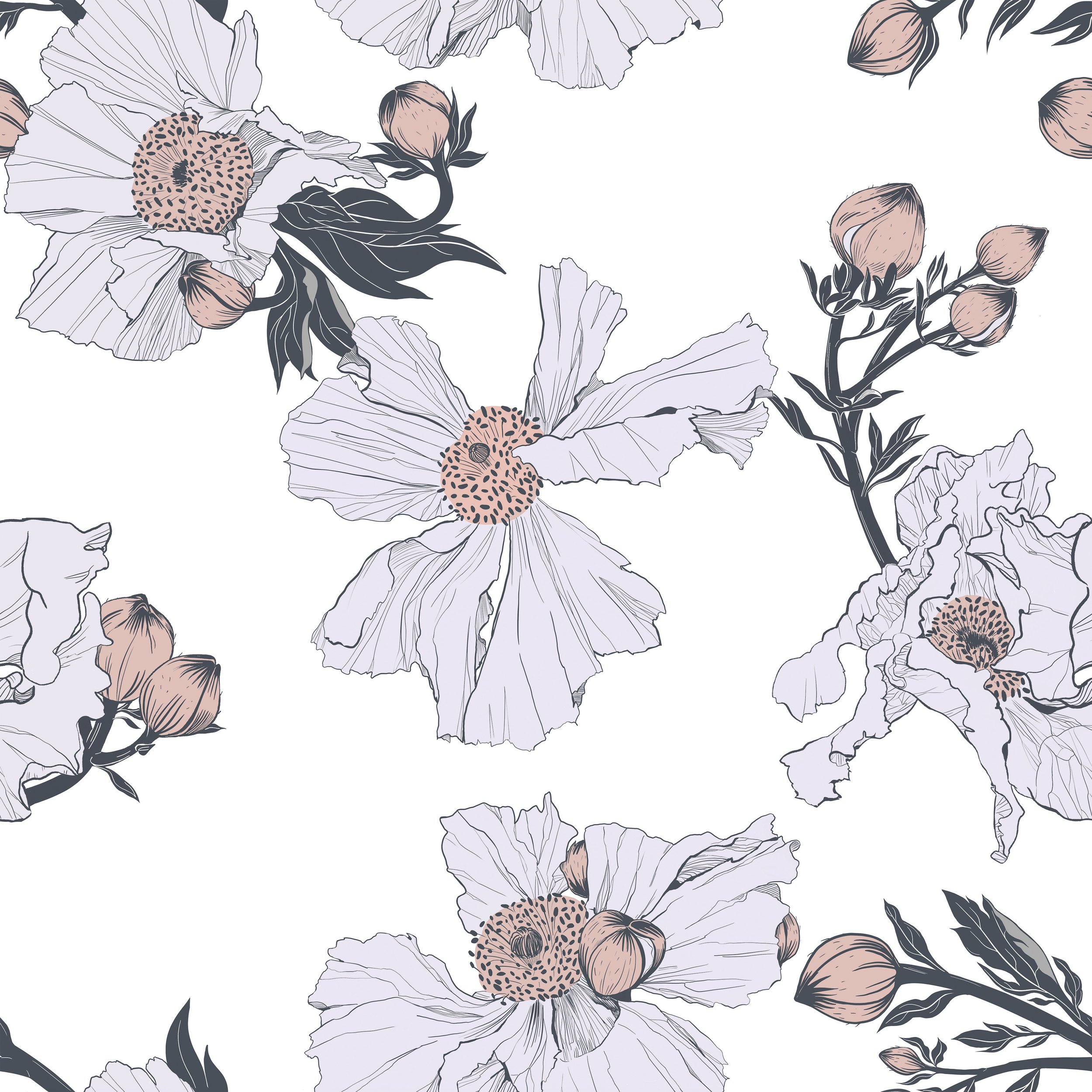This hand-drawn floral artwork, resembling a sophisticated wallpaper print, features an arrangement of Matilija poppies against a solid white backdrop. Dominated by hues of black, white, and pale tans, the piece is accented with subtle greens. Central to the composition are white-petaled flowers, each with a pale tan center filled with seeds. Interspersed among the blooming flowers are several closed buds on dark green stems, hinting at future blossoms. These stems, darker yet tinged with green, suggest depth against the stark background. The repetitive nature of these floral images, with their distinct white petals and pale centers, lends the piece a textile-like quality, making it reminiscent of elegant, evening mauve wallpaper.